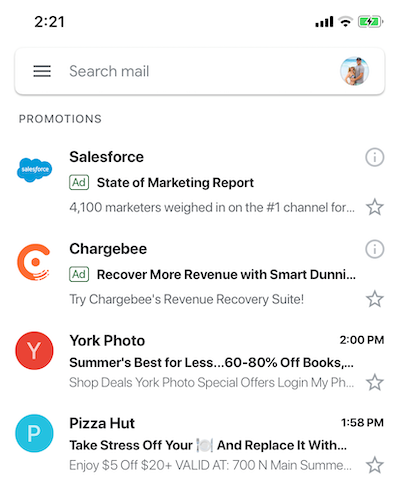A screen capture of a smartphone displays the time as 2:21 PM, with full reception indicated by 4 bars and a WiFi connection at half strength. The phone is currently charging, denoted by a small lightning bolt icon within the battery symbol. The email app's search bar reads "Search mail," suggesting it's open to Gmail. At the top of the screen, various advertisements are visible, including:

1. An ad for Salesforce’s "State of Marketing Report," noting that 4,100 marketers provided insights on the top marketing channels.
2. An ad for ChargeBee’s revenue recovery suite, promoting effective revenue recovery strategies.
3. A York Photo ad promoting summer sales with 60-80% off books and special deals.
4. An ad for Pizza Hut offering $5 off orders of $20 or more, valid at their location on 700 North Main Street.

These ads point towards a Gmail interface, given the nature and layout of promotional content commonly seen in such accounts.